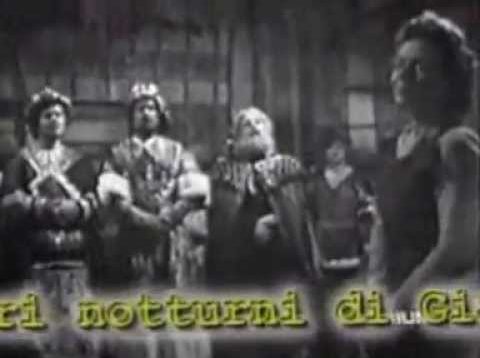The image depicts a somewhat faded, black and white scene that appears to be a screenshot from a television show set in medieval times, featuring luxurious clothing and crowns, suggestive of nobility or royalty. The people, mostly dressed in medieval-style costumes, are primarily positioned in the center of the frame within a large antechamber. Notably, a woman stands prominently in the foreground on the right-hand side, her body turned to the side as she looks straight ahead. Behind her, along the back wall, are four men: a younger man with dark hair on the left, a slightly older man with folded arms and dark hair next to him, an older gentleman with white hair and a beard, and another younger man or boy to his right. The image includes text at the bottom in fuzzy yellow lettering, which appears to be in a foreign language, possibly Italian, and includes words like "Natarni D.G."